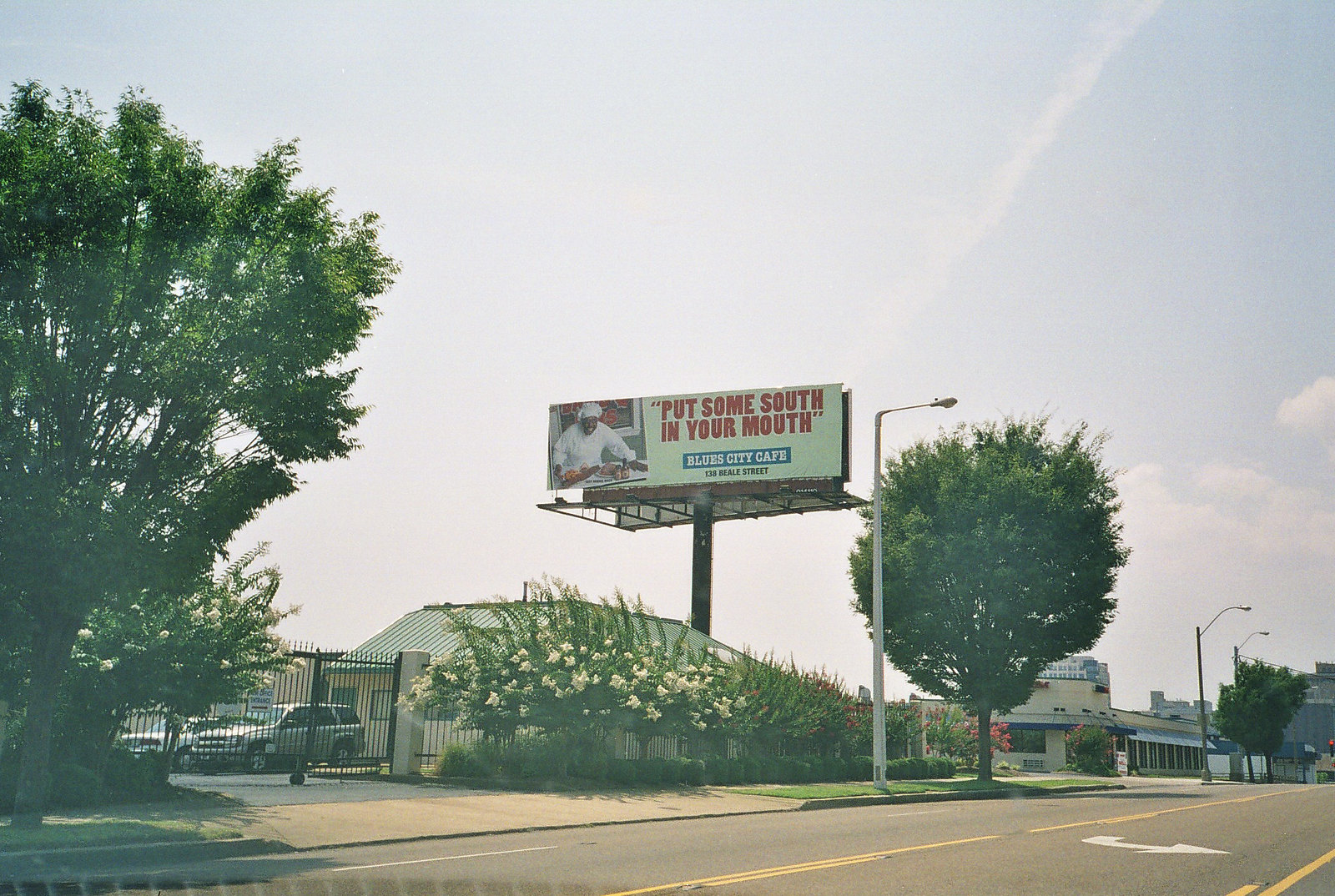The image captures a roadside billboard nestled between two distinct businesses. On the right side of the image, a building extends from the lower right corner, stretching to the far right, gradually widening as it approaches the road. The road itself spans from the left corner to the far-right corner, creating a clear thoroughfare. On the bottom left side of the image, a tree is situated alongside the road, adding a touch of nature to the scene. Adjacent to the tree, on the right, a closed gate marks the entrance to a business located just beyond it.

The billboard, prominently positioned and supported by a pole behind the aforementioned building, features a vivid advertisement. On the left-hand side of the billboard, a picture of a chef is displayed, accompanied by an intriguing caption: "Puts themselves in your mouth." The billboard's pole is discreetly visible behind the building, creating a seamless yet striking visual in the overall setting.